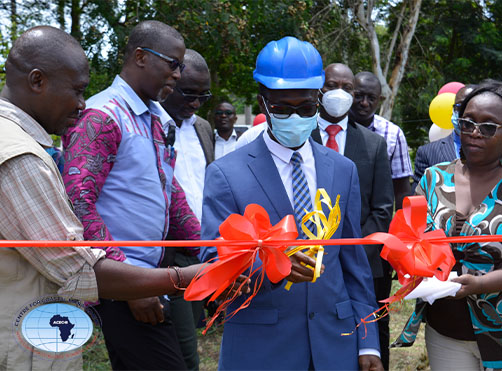In this image taken outdoors on a partially sunny day, we see a ceremonial ribbon-cutting event taking place in Africa, indicated by a logo with a globe that says "Africa" in the bottom left corner. Centrally positioned is a man in a blue suit, white shirt, and blue-striped tie, wearing a blue hard hat and a surgical mask, about to cut an orange ribbon. He also holds a yellowish ribbon in his hand. Surrounding him are several people, including a woman in sunglasses and a blue top with white trousers, and three men: one in a tan shirt with rolled-up sleeves, another in a blue shirt with red sleeves and black trousers, and a third in a white shirt with sunglasses. The background features a forest with thick green foliage and scattered balloons, suggesting a celebratory atmosphere in a warm climate. Although there is text present in the image, it is too small to read.